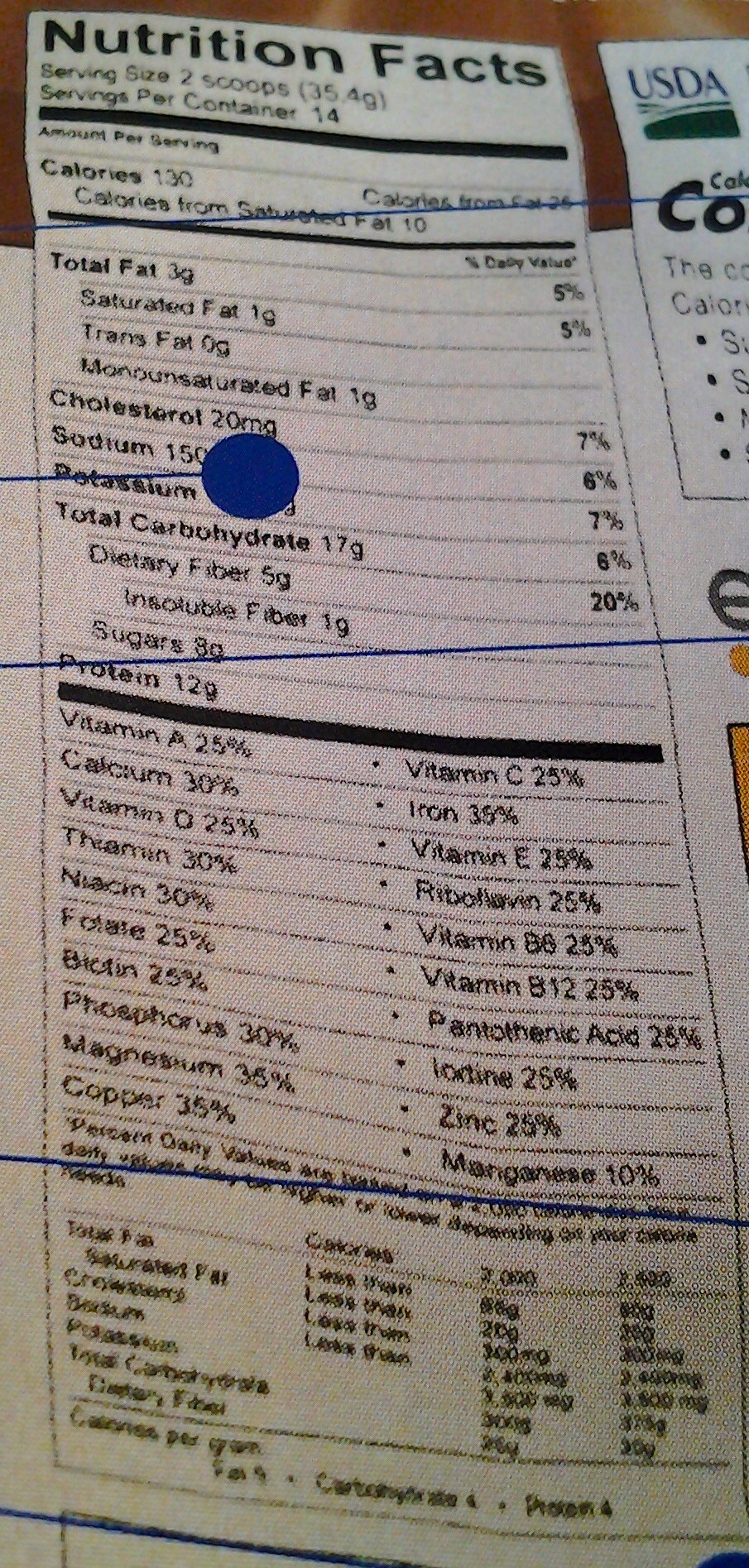A somewhat grainy photo captures the Nutrition Facts panel of a food item's packaging. The panel features several thin, royal-blue lines running horizontally across it. In particular, one prominent blue dot stands out, connected to the edge of the image by a blue line.

The serving size is specified as two scoops. Key nutritional details are as follows: 
- Calories: 130 
- Total Fat: 3 grams 
  - Saturated Fat: 1 gram
  - Monounsaturated Fat: 1 gram
- Cholesterol: 20 milligrams
- Sodium: (value obscured)
- Total Carbohydrate: 17 grams 
  - Dietary Fiber: 5 grams 
  - Insoluble Fiber: 1 gram
  - Sugars: 8 grams
- Protein: 12 grams

The panel also includes a detailed breakdown of the vitamin content, positioned below the macronutrient information.